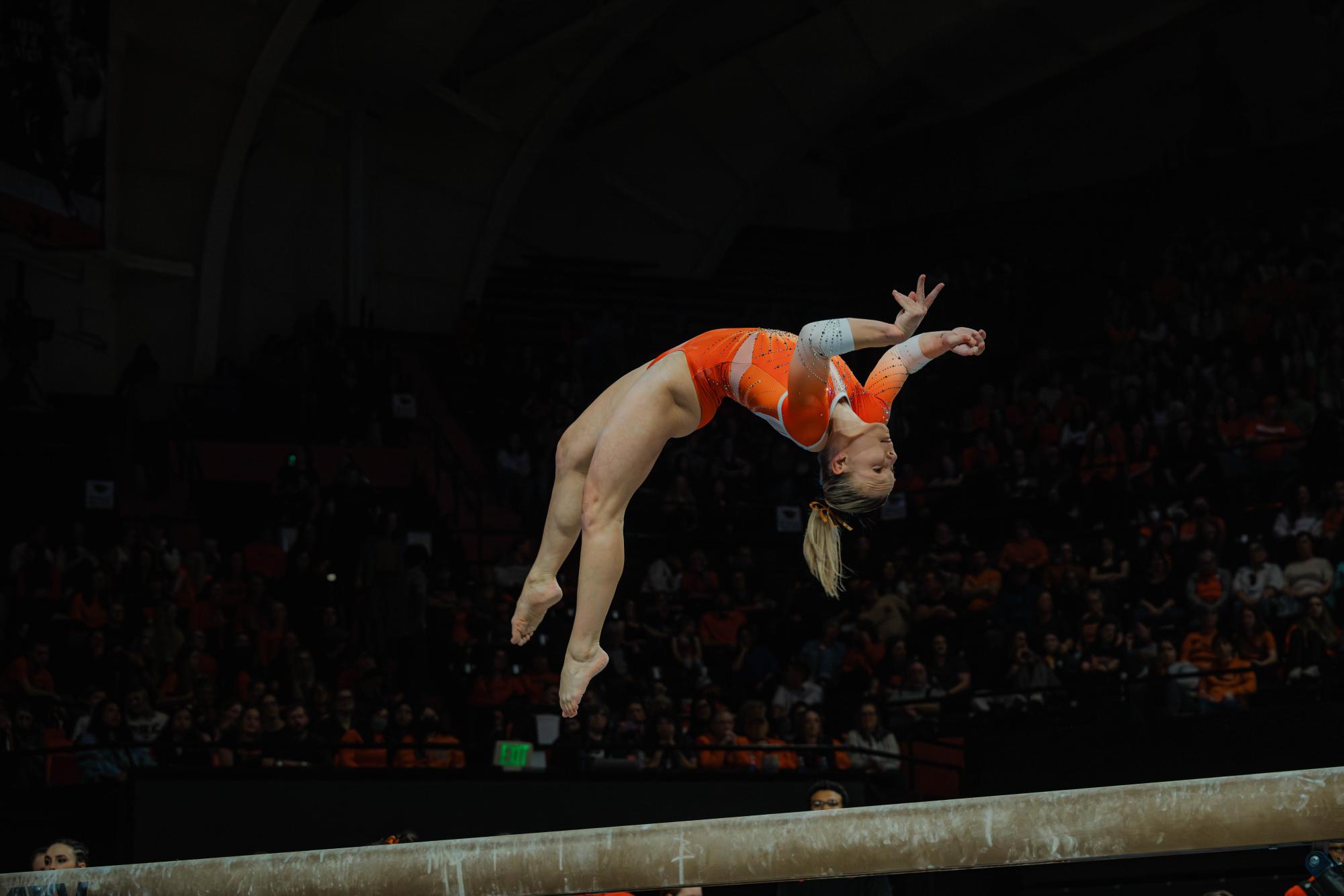The image captures a thrilling moment at a gymnastics tournament. Dominating the center is a fair-skinned female gymnast, suspended in mid-air as she executes a backflip. Her body is arched gracefully, with her hands poised above her head and her blonde hair, tied in a ponytail, cascading backwards. Dressed in a striking orange leotard with white and glitter accents, she has wristbands or elbow bands but no footwear, revealing toned legs and feet.

Below her, the brown balance beam, streaked with white chalk marks from previous gymnasts, stretches horizontally across the frame. This beam serves as the focal point of her performance. The background, though dimly lit, reveals a crowded stadium with spectators intently watching the gymnast's routine. High ceilings with visible steel beams add to the grandeur of the venue, emphasizing the extensive height of the performance area. The observation of the audience in shadowy stands and the structural details of the venue underline the scale and intensity of the live event.